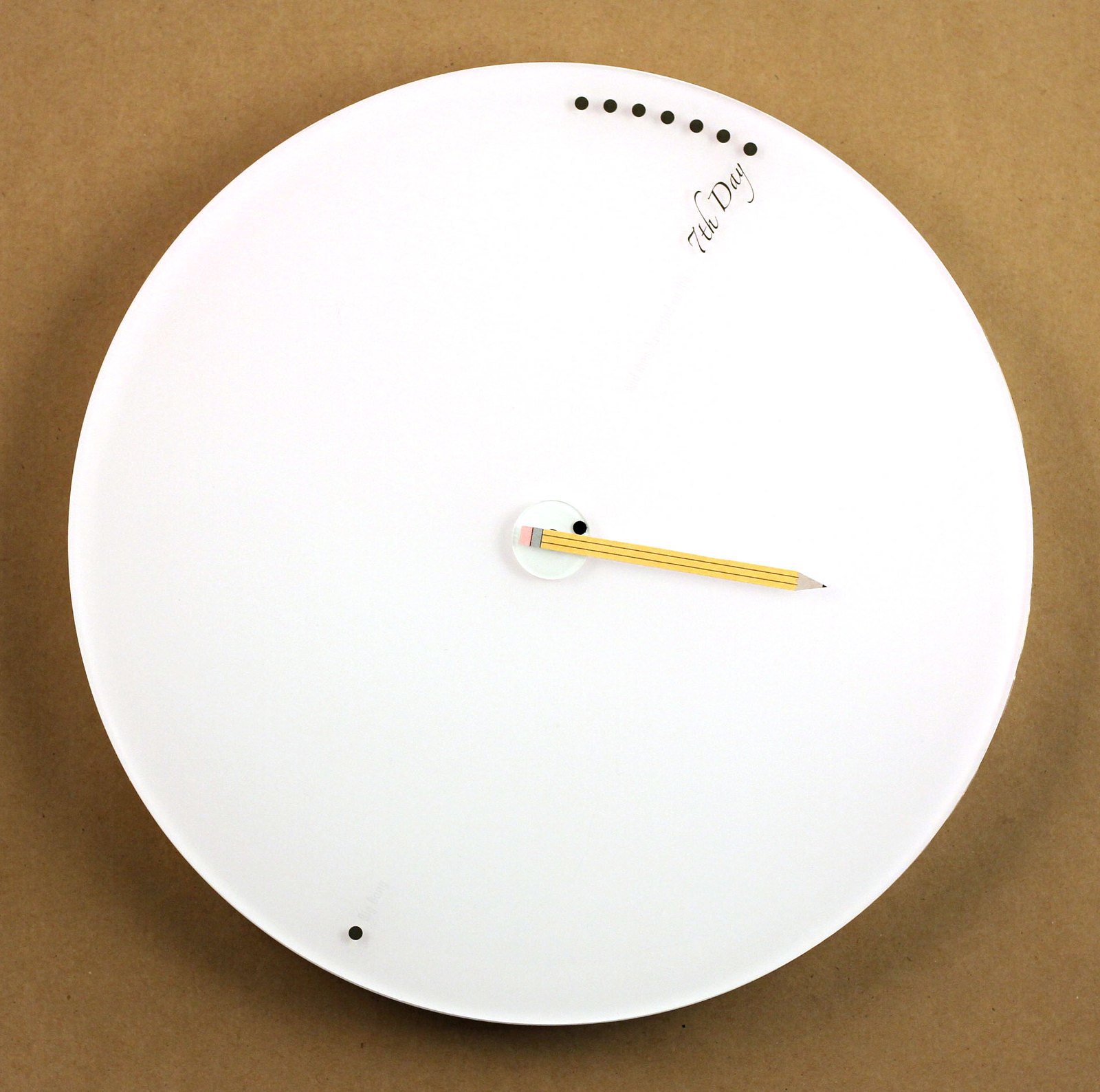On a brown backdrop, the image features a large white circle that resembles the face of a clock. At the center of the circle is a cardboard cutout or drawing of a number two pencil, characterized by its yellow body with center lines, an orange-pink eraser, and a sharpened graphite point. The pencil is angled slightly downward towards the right, mimicking an hour hand on a clock. Adjacent to this pencil "hand" is a single black dot. 

On the left side, also slightly downward, there is another black dot. To the right and slightly upward, there is a sequence of seven black dots arranged in a row. Beneath these seven dots, the text "seventh day" is inscribed, suggesting that the image may be a conceptual clock used for counting days rather than minutes or hours.